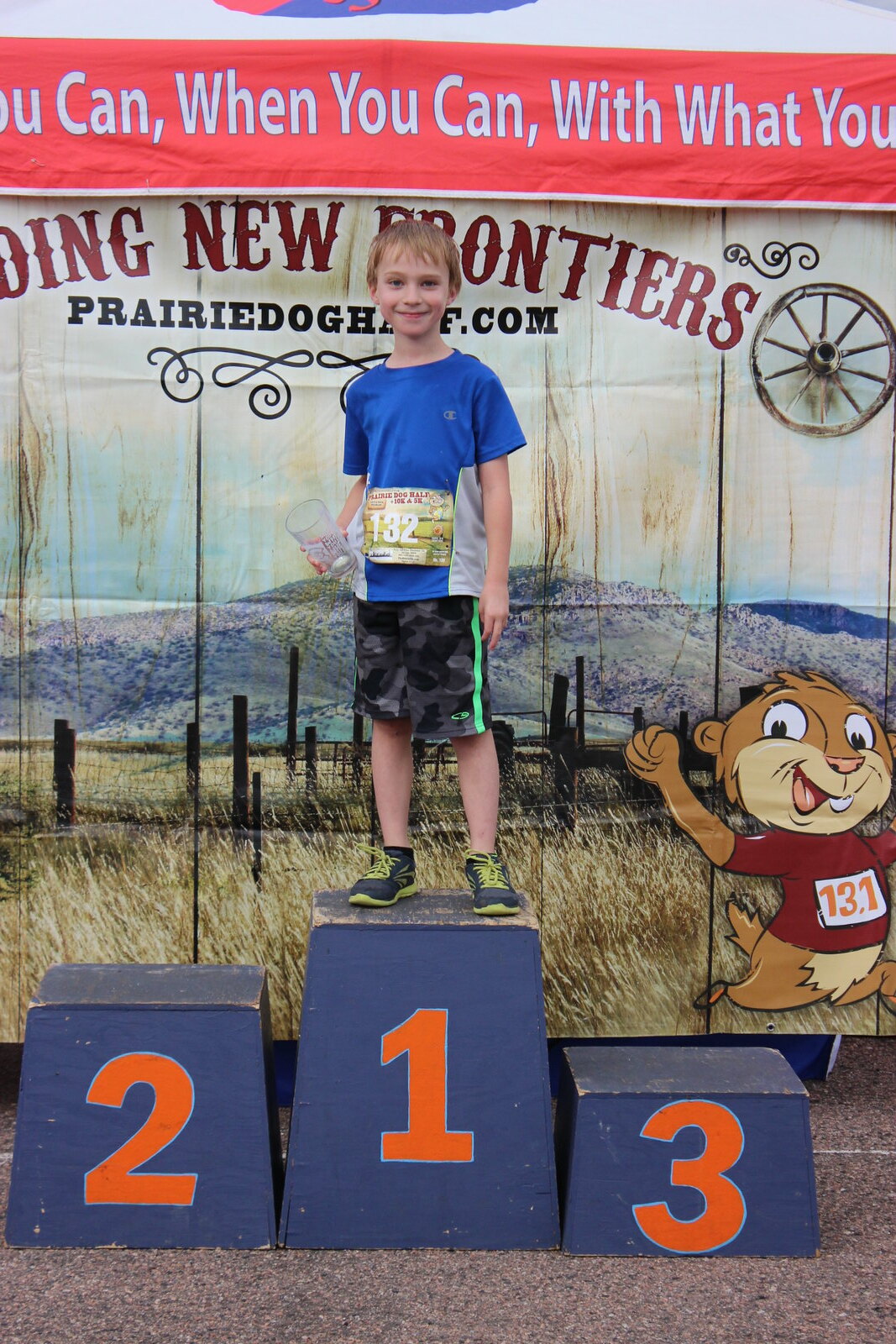This image captures a young blonde-haired boy, likely around eight or nine years old, standing proudly on the first-place pillar of a blue podium marked with the number 1 in orange. The second and third-place pillars remain empty. He appears to have just completed a race, possibly the Prairie Dog Half Marathon, as suggested by his race bib numbered 132. The boy is dressed in a blue athletic shirt, black camo-patterned shorts, and black and green sneakers. He holds an empty plastic cup in his right hand, possibly from the event. Behind him is a painted wooden backdrop depicting a prairie scene with a fence and rolling hills, adorned with a red banner partially displaying the words, "when you can, with what you." Another prominent feature of the backdrop is a red-shirted prairie dog mascot, wearing a bib labeled 13.1, indicative of a half marathon. The backdrop also includes the text "New Frontiers" in red, and "PrairieDogHalf.com" below it.